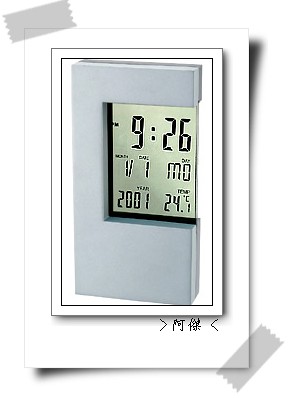The image depicts a meticulously detailed drawing of a digital clock positioned at the center of a white card, about the size of a greeting card. The white card is taped to a white surface with what appears to be digital representations of translucent gray tape, placed at the upper left and lower right corners, with edges that are ragged. Surrounding the central gray clock illustration, which exhibits a 3D, tilted-outward appearance, is a rectangular frame formed by two black outlines with a white space in between, mimicking the look of a picture frame.

The clock itself is a sleek, gold-ish or gray piece with a C-shaped body encasing a thin, glass display panel. The time displayed is 9:26 AM in bold, black LED-style numbers. Additional information shown on the clock includes the date "1/1," the day "MO," the year "2001," and the temperature "24.1°C." The image also contains some Asian characters, possibly Japanese, and a faint black shadow around the card, enhancing the drawing's sense of depth and realism. Moreover, there are subtle details of shading within the squares, enhancing the overall three-dimensional effect of the illustrated clock.